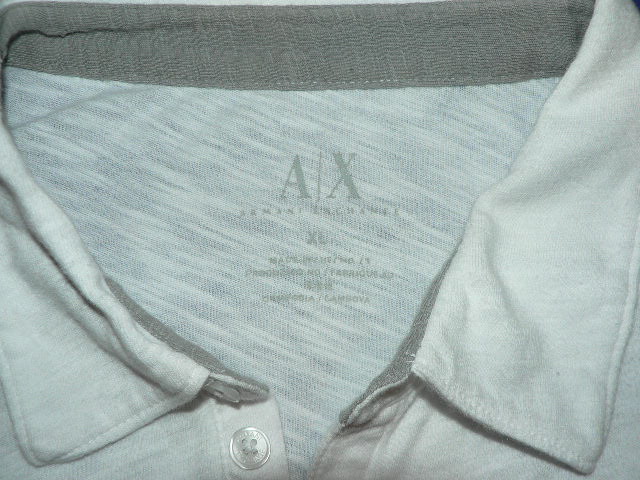This photograph, taken indoors during the daytime, offers a close-up view of the upper portion of a knit collared pullover shirt. The frame focuses on the top two buttons and the collar, providing a detailed perspective on these elements. The collar's inside exhibits a distinct gray color, contrasting subtly with the shirt's overall white hue. The buttons are small, white, and semi-transparent. At the back of the collar, there's a zoom-in on the shirt tag, which reveals the brand "AX Armani" and the size "Extra-Large," though the tag's print appears quite faded and partially illegible. The image composition emphasizes the texture and structure of the garment, highlighting the quality and subtle intricacies of the fabric.